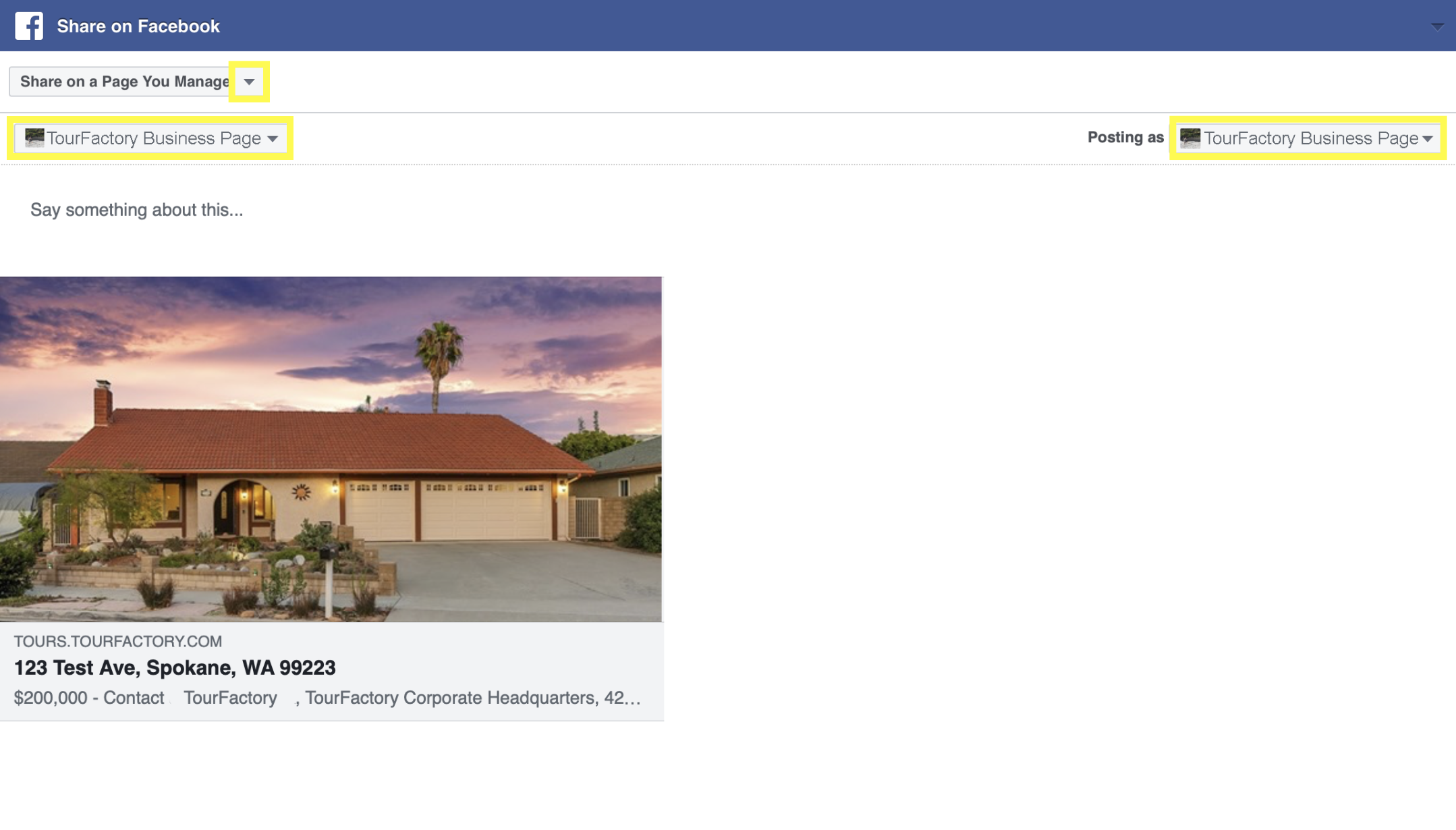This detailed caption describes the image of a Facebook page admin panel with multiple elements highlighted for emphasis:

**Image Description:** The image showcases the admin panel of a Facebook page. At the very top, there's a blue header bar featuring the Facebook icon on the left side, followed by the text "Share on Facebook." Below this header, a significant part of the interface is filled with a gray box labeled "Share on a Page You Manage," which includes a yellow box edited around the drop-down options within it, emphasizing this section.

Directly beneath this gray box, there is a business page titled "Tor Factory Business Page" displayed within a drop-down box, which is also highlighted with a red and yellow box for emphasis. To the far right of this section, you can see the words "Posting As," accompanied by another drop-down box selecting "Tor Factory Business Page," again highlighted by an edited yellow box.

In the bottom left corner of the panel, the prompt "Say something about this..." invites users to add commentary. Below this, there is a listing featuring a photo of a house, including the website address, the physical address of the house, the price, and contact information directing inquiries to "Tor Factory." The company's contact details, including the Tor Factory address, are also provided at the bottom of this listing.